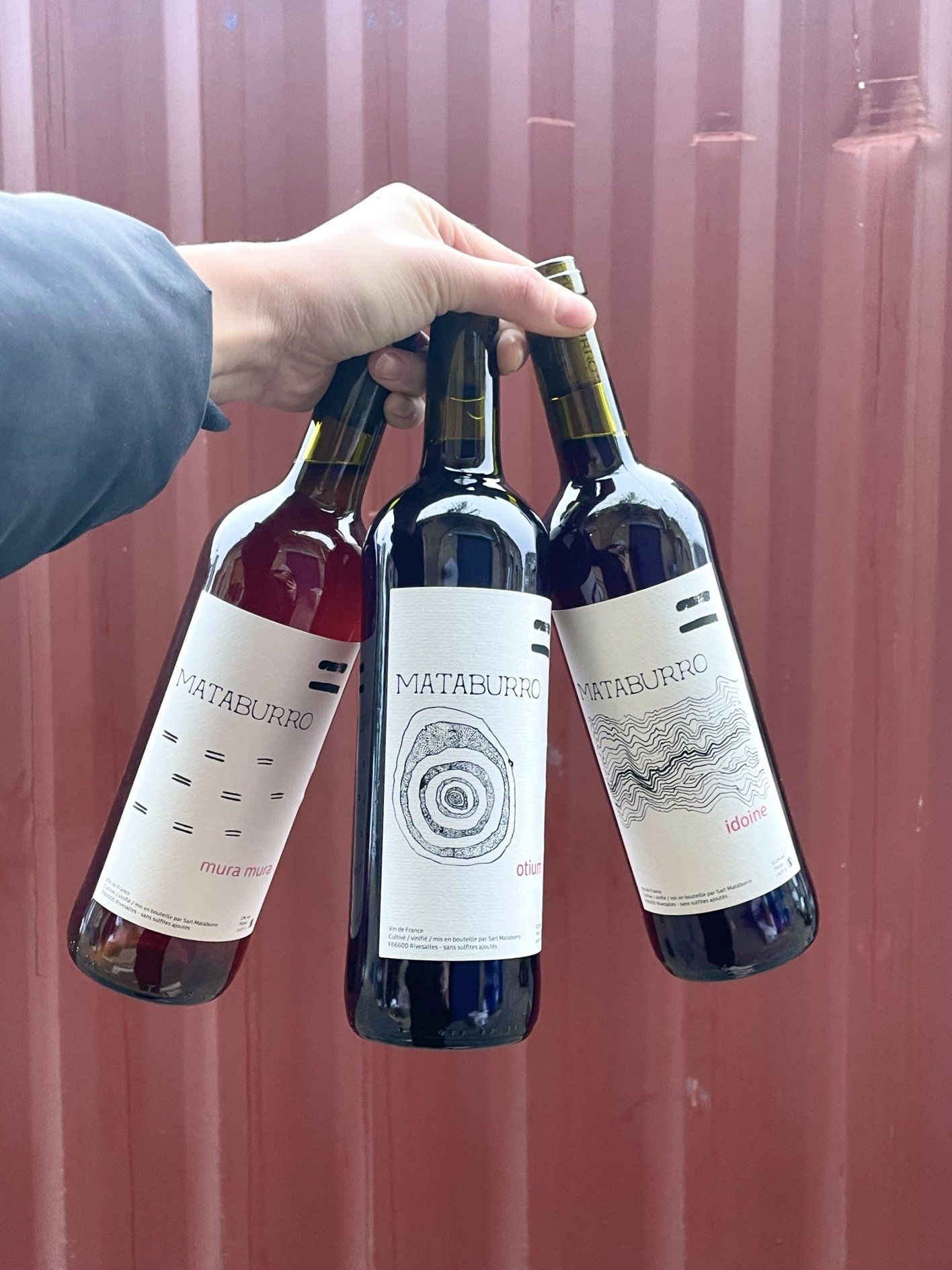In this color photograph, we see a left hand extending from the left side of the frame, holding three wine bottles. The person, whose body isn't visible beyond their arm, is wearing a gray jacket. The white hand firmly grips the bottle tops, demonstrating a confident hold. The bottles—each with a cylindrical shape and white labels—display the brand name "Mataburo." Each label features unique illustrations: the leftmost bottle has concentric circles, the middle one is darker with an unidentified design, and the rightmost bottle shows a wavy pattern with "Mataburo" text prominently at the top and additional red text near the bottom. The background is filled with a red or burgundy corrugated metal wall, adding a vivid, textured contrast to the composition.